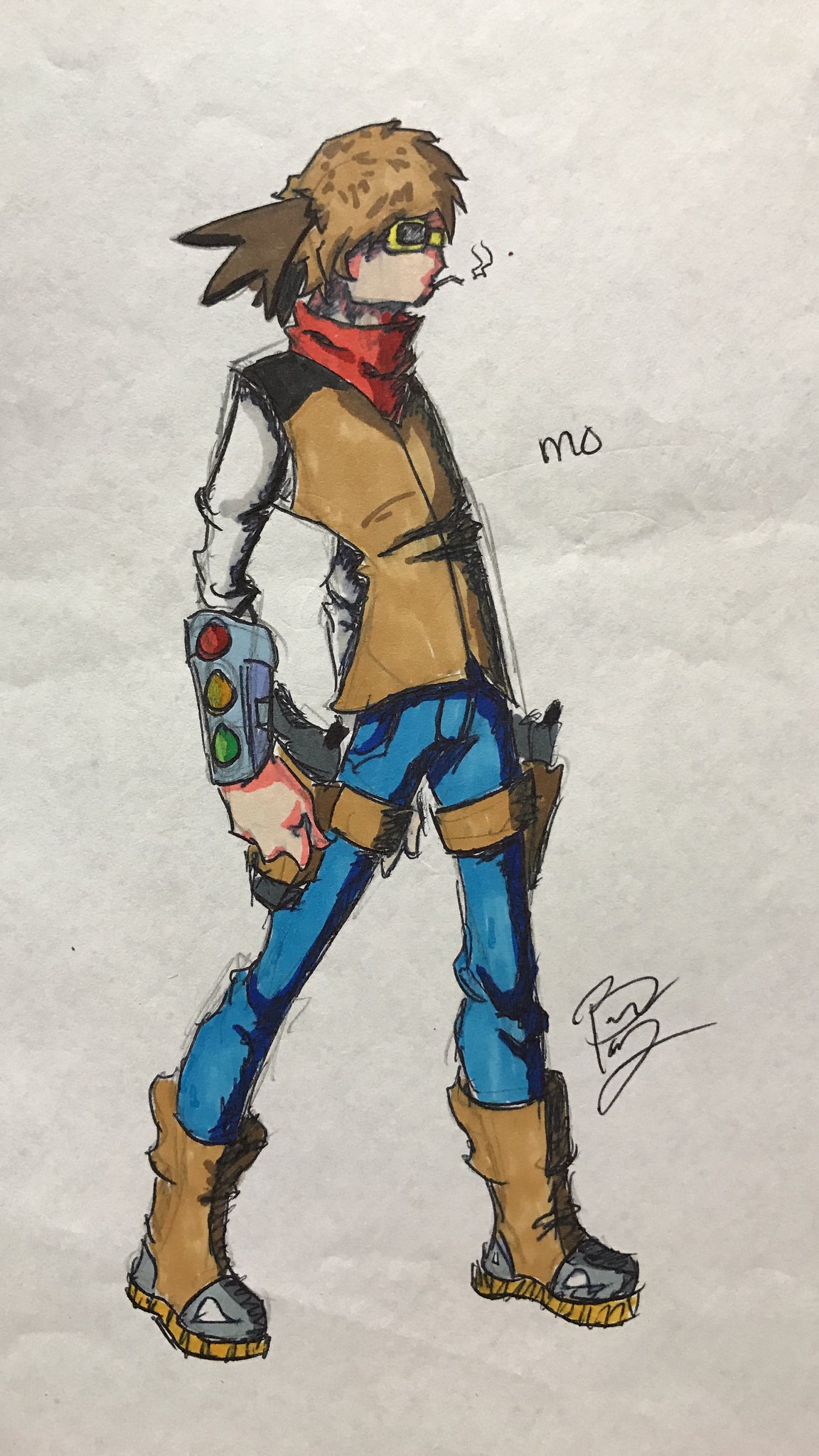This is an image of a detailed drawing of a male character, somewhat resembling an anime or cartoon style. The character has light brown hair and is dressed in blue pants along with light brown, gray, and black boots. He is equipped with a holster strapped around each thigh, each containing a gun. The character dons a long-sleeved shirt and a brown vest. Over his right wrist and lower arm, there's a covering that is gray, adorned with three circular lights in a sequence from bottom to top: green, yellow, and red, resembling a stoplight. He accessorizes with a red bandana tied around his neck and is sporting yellow glasses. A lit cigarette is held in his mouth. The illustration is on white paper, captioned with "M.O." and signed at the bottom right.